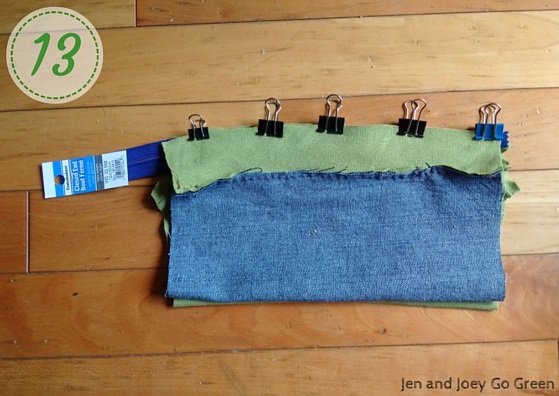This photograph captures a detailed setup for a sewing project laid out on a natural wooden surface. Central to the image is a green piece of cloth layered over a blue piece of cloth, both held together by five clips. Four black clips secure the fabric, with three being uniform in size and the one on the far left being considerably smaller. A distinctive cyan clip stands out at the far end. In the top left-hand corner, the number 13 is prominently featured inside a beige circle adorned with green dashes. The bottom right-hand corner has black text that reads, "Jen and Joey, go green." This staged scene likely represents a preparatory step in a sewing pattern assembly, emphasizing the final stages with a visible zipper and indicating the project belongs to "Jen and Joey Go Green."